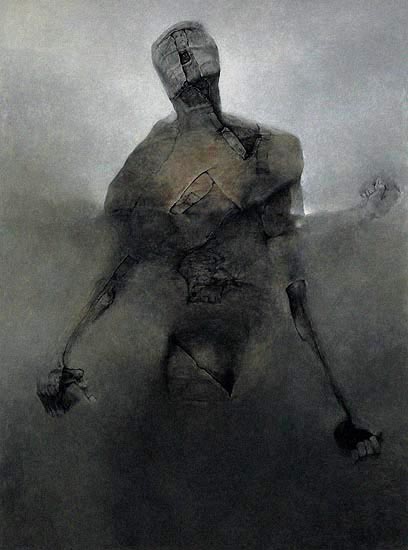This is a surrealistic, symbolic painting by Zdzislaw Beksinski, featuring a human-like figure composed of rock and straw-like elements. The overall color palette is dominated by various shades of gray, ranging from light to nearly black. The figure occupies the central part of the image, which is in portrait orientation. Its head, appearing to be a stone with slits for eyes and an open mouth, is tilted up and to the side as if crying out or yelling. The background is a gradient of light gray on the top, becoming darker towards the bottom, and features a light source illuminating the head and shoulders of the figure. The figure's upper body, including its broad shoulders and torso, appears to be made of rock, with sinewy, stick-like arms ending in robotic-looking fingers. The lower part of the figure fades into a dark gradient, obscuring any details of the legs. The setting appears to be outdoors, with a dark cloud-like sky adding to the eerie, non-realistic atmosphere. There is no text in the image, and the painting expertly captures a haunting, otherworldly presence reminiscent of a man standing and looking up at the sky, wrapped in bandage-like materials.